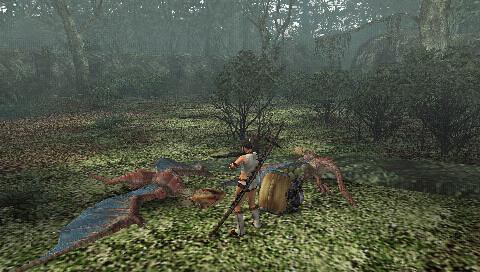In this grainy video game screenshot, the foreground features a white male character standing in an open, but lush and dense forest brimming with trees, bushes, and green leaves covering the ground. He wears knee-high white boots, white shorts trimmed with leather, and leather armbands, with a dark-haired ponytail. Over his back, he carries an oversized weapon—which seems to be either a giant bow, long spear, or katana—extending well above his head. This figure is possibly shirtless, although some descriptions suggest a white tank top. The character stands over a slain creature lying on the ground to the left, described variably as a 'Raptor' or 'dragon baby' with long, pterodactyl-like wings, exhibiting reddish-pinkish hues. To his left, there seems to be a large sack, while another similar creature can be seen in the background to the right. The ground is littered with leaves and sparse small trees, with a rock embankment curving around the scene from the far left to the right, emphasizing the setting's rugged and natural environment. The image lacks any user interface elements, reinforcing its focus on the immersive, ancient hunt-like atmosphere.